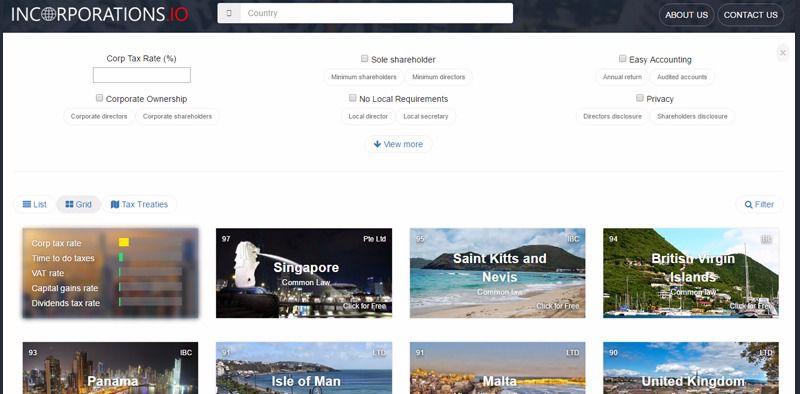This is a detailed screenshot of the Incorporations.io website, displaying its main interface. 

**Header and Logo:**
- The website features a dark blue header with a thicker top bar, giving it a structured appearance.
- On the upper left-hand corner, the Incorporations.io logo is prominently displayed in bright text. Notably, the first "O" in "Incorporations" is designed as a globe symbol, while ".io" is highlighted in red text.

**Search and Navigation:**
- Centrally positioned on the page is a search bar labeled "Country," intended for users to input their search criteria.
- To the right of the search bar are two clickable buttons: "About Us" and "Contact Us."

**Tax and Corporate Options:**
- Directly below the search bar, users are provided with a field to enter the "Corporate Tax Rate" percentage.
- Adjacent to this field are options related to corporate structure, including "Sole Shareholder," "Minimum Shareholders," and "Minimum Directors."
- Further to the right, there is a clickable option for "Easy Accounting," indicated by a checkbox. Alongside this, users can access information on "Annual Returns" and "Audited Accounts."

**Corporate Ownership and Requirements:**
- Below the "Corporate Tax Rate" input field, there is a section for "Corporate Ownership" where users can specify options, including "Corporate Directors" or "Corporate Shareholders."
- Beneath the "Shareholder" section in the middle, there's a "No Local Requirements" segment, which can be toggled to include "Local Director" and "Local Secretary."
- To the right of these sections, under "Privacy," options for "Director's Disclosure" or "Shareholder's Disclosure" are displayed.

**Additional Features:**
- At the center bottom of the page, there's a "View More" button accompanied by a downward-pointing blue arrow.

**Images and Filters:**
- The page also features a gallery of eight images representing different countries, which can be sorted by "List," "Grid," or "Tax Treaties," with the "Grid" view currently selected.
- A "Filter" button is situated to the right of the sorting options.

**Country-Specific Tax Information:**
- Starting with the first image, it appears highlighted and displays various tax-related metrics such as "Corporate Tax Rate," "Time to Do Taxes," "VAT Rate," "Capital Gains Rate," and "Dividends Tax Rate."
- The following entries represent specific countries: "Singapore (Common Law)," "St. Kitts and Nevis (Common Tax)," "British Virgin Islands (Common Tax)," and then "Panama," "Isle of Man," "Malta," and "United Kingdom," though the lower portions of these images are not fully visible.